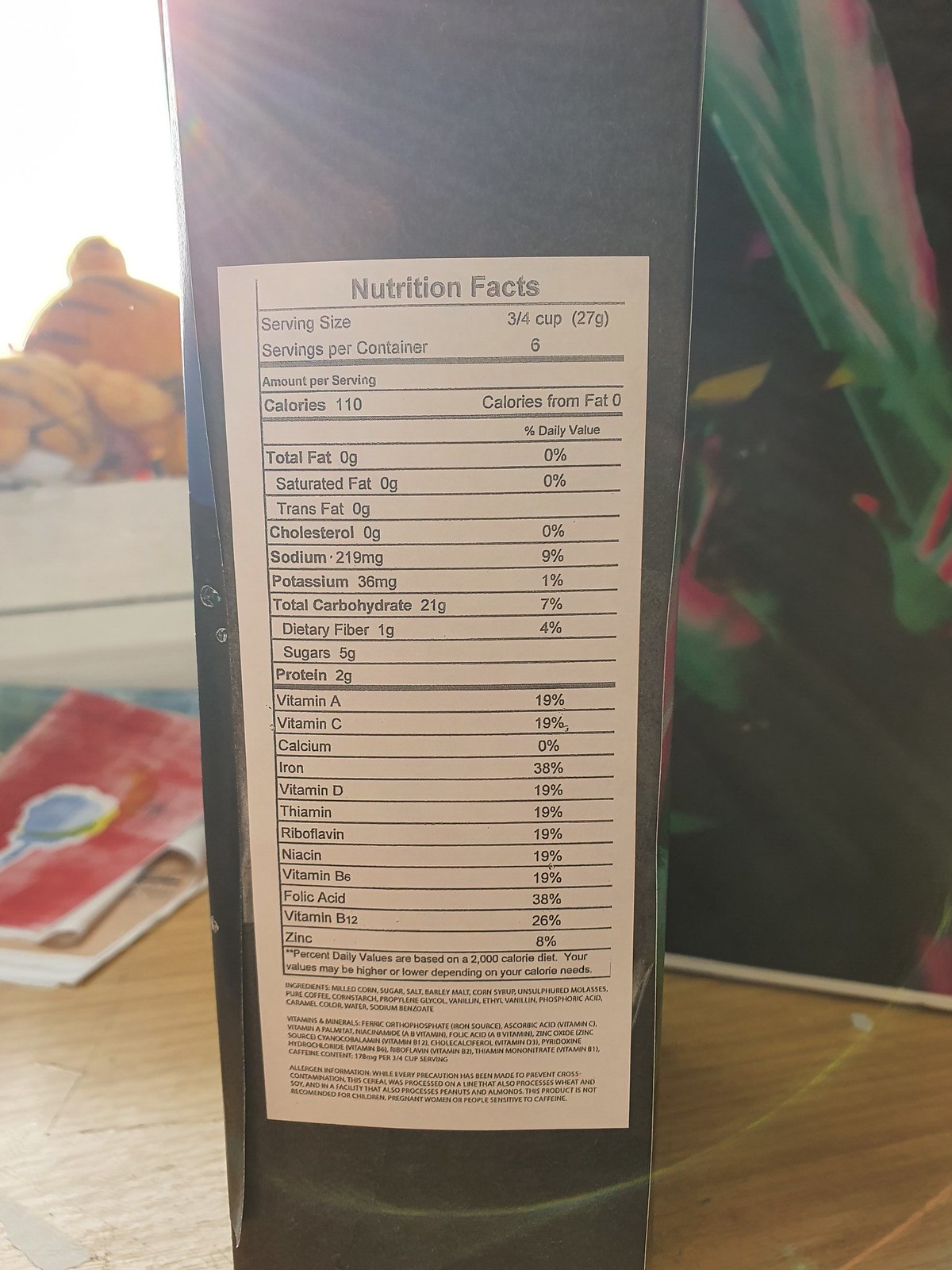Captured in the photograph is a black rectangular box positioned on a brown wooden tabletop, showcasing its nutrition label prominently on the side. The label, featuring white text on a black background, provides nutritional information in a clear, legible font. 

To the left of the box lies a neatly folded newspaper, topped with a mostly-red picture bordered by a bluish circle outlined in white. Behind these items, a shelf is visible, housing a Garfield stuffed animal faced down. On the right-hand side of the image, there is a black-painted wall or window shade adorned with an intricate design of green and pink leaves, interspersed with yellow flowers. Light reflections are noticeable at the bottom right corner of the photograph, adding a subtle sheen to the captured scene.